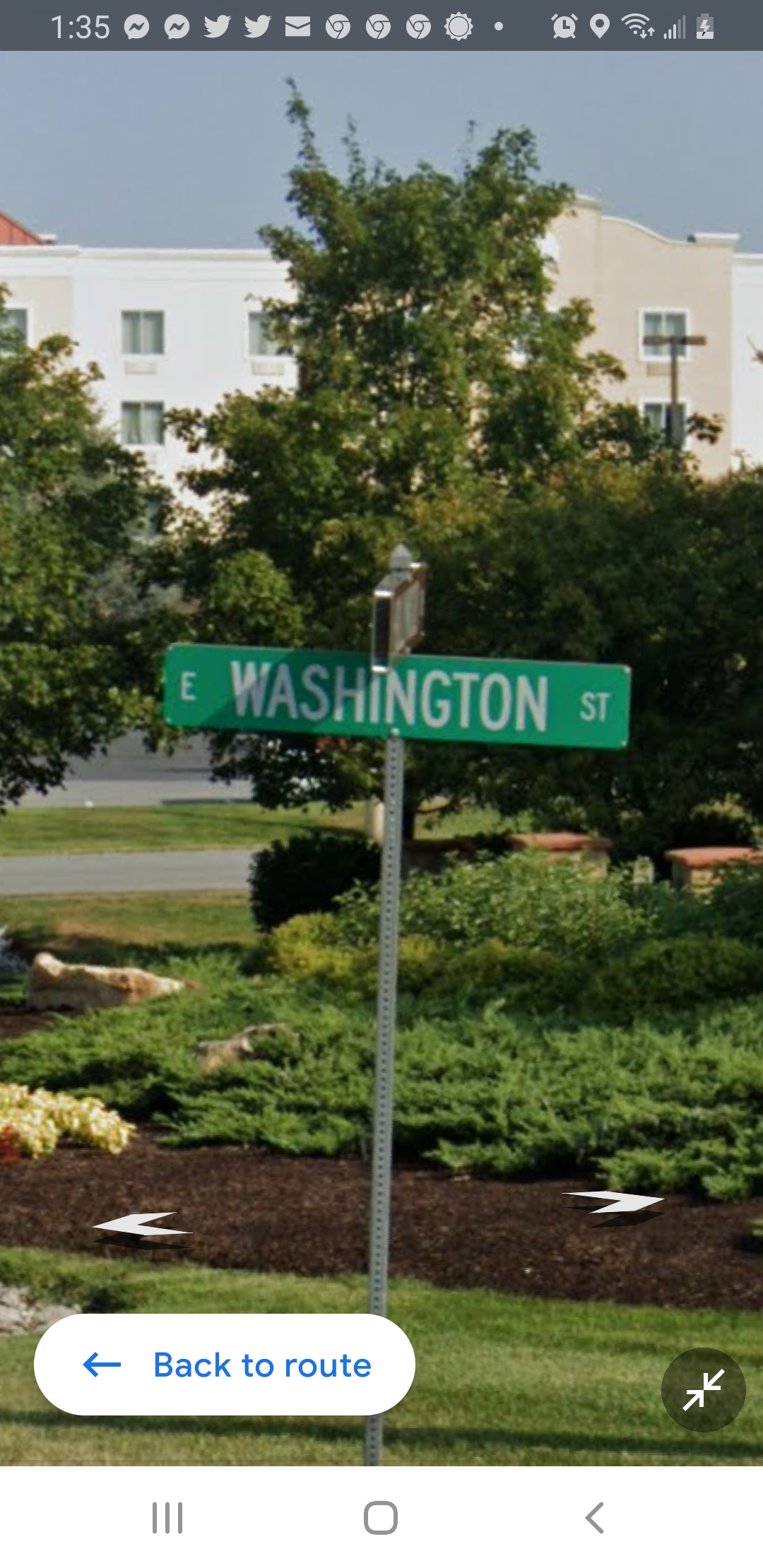This vertical photograph appears to be a screenshot from a smartphone. At the very top, there is a dark gray status bar displaying the time as 1:35 in the upper left-hand corner, along with various icons including message alerts, tweet notifications, a mailbox icon, and possibly three Chrome browser icons, among others.

The central image depicts an outdoor scene featuring a street sign labeled "East Washington Street," intersecting with another street whose name is obscured as it faces away from the viewer. Prominently in the middle, there is a traffic circle or a wide median, surrounded by lush trees. In the background, a large, white building is visible.

In the lower left-hand corner of the screenshot, a clickable icon reads "Back to Route" in blue text on a white background, accompanied by a blue arrow pointing left. At the bottom right, there is a zoom control icon. Superimposed on the traffic circle greenery are left and right carets, characteristic of GPS navigation interfaces, providing directional instructions.